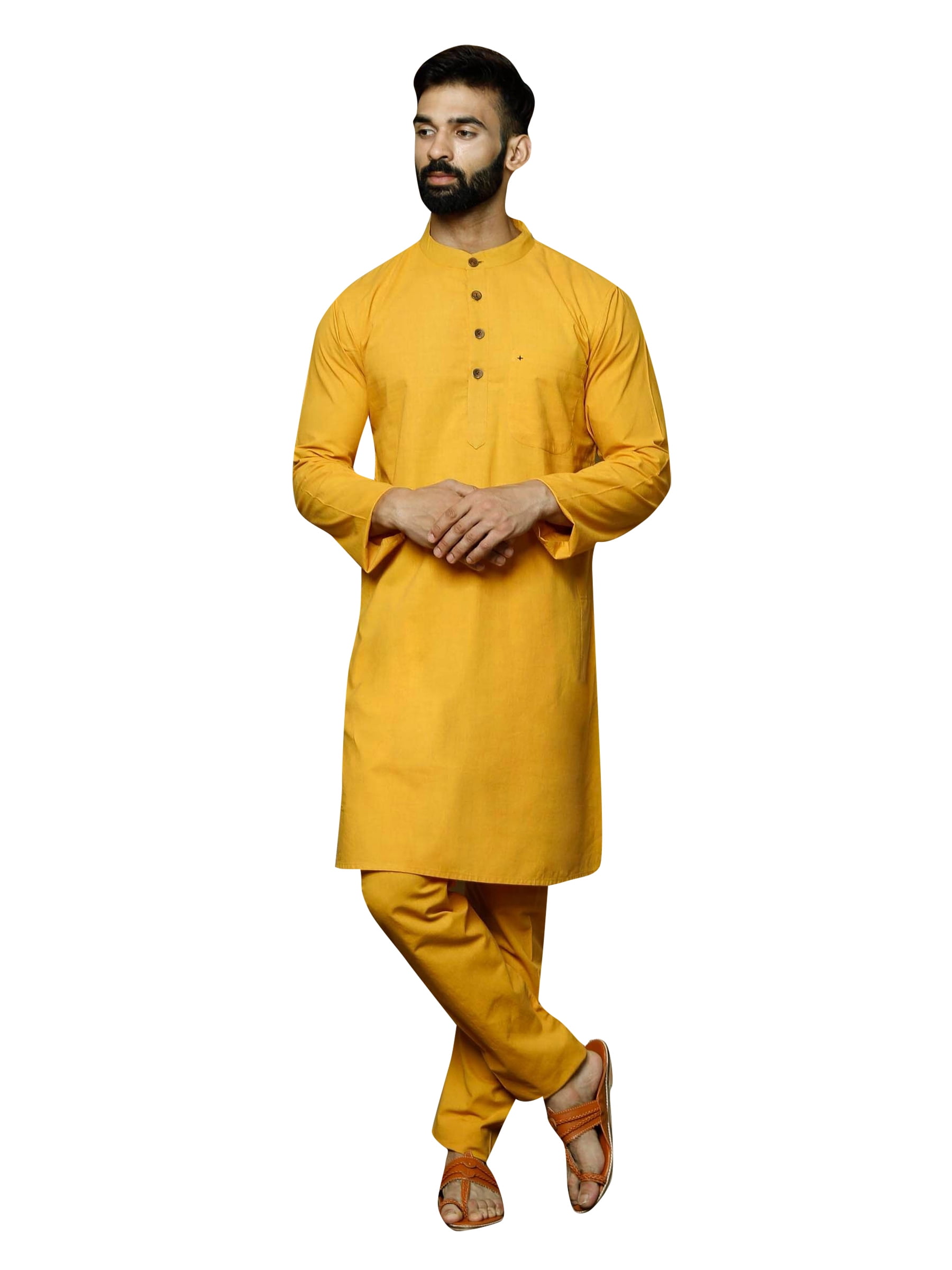This is an image of a middle-aged man with olive skin, dressed in a stylish all-yellow ensemble. The man, who appears to be of Middle Eastern descent, has thick black hair, a well-groomed full-trimmed beard, and a matching mustache. His expressive brown eyes are directed slightly to his right, giving him a contemplative look as he stands. He is clad in a long yellow tunic that extends to his knees, featuring four buttons descending from a priest-like collar down to the chest area. Beneath the tunic, he wears matching mustard yellow pants that go down to his ankles. His feet are shod in reddish-orange thong sandals, which reveal all of his toes and have flat soles.

In his pose, the man stands with his right leg crossed over his left, with his toe touching the ground and heel raised, displaying his footwear. His hands are clasped together at his midsection, right arm resting over his body while the left hand gently holds the right. The background of the image is entirely white, making it appear as if the man has been cut out and placed on a blank canvas, possibly for an advertisement showcasing his distinctive attire.